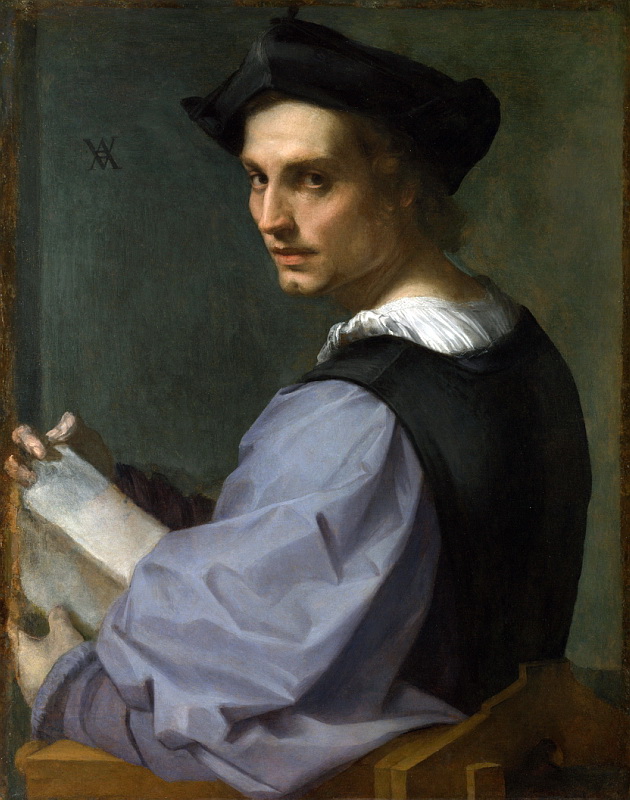The image depicts a detailed Renaissance-style painting or drawing of a young man, likely a scholar, seated on what appears to be a wooden chair or bench. The man, who has a light complexion, is wearing a distinctive outfit comprising a blue bodice with a puffy white undershirt and a black vest. He is also donning a black hat typical of the 17th century. His face, turned to look at the viewer over his left shoulder, portrays a neutral expression, with both eyes visible and a prominent nose, devoid of facial hair. 

In his hands, he holds an object that might be a book, scroll, tablet, or piece of paper, with his right hand resting on top and the left hand cradling the bottom. The background features a dark color, described variably as blue or greenish-gray, with two X symbols etched on the upper left side. The chair he sits on is brown, possibly wooden. In the foreground, there appears to be a logo resembling an inverted 'V' or an 'A', possibly a signature, adding a distinct element to the scene. The image is richly colored, featuring shades of white, black, gray, light blue, brown, and green.